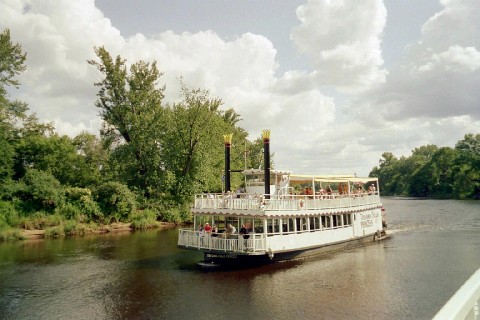This photograph captures a white, two-level steamboat navigating a narrow, brownish-colored river flanked by green trees on both sides. The steamboat, with a white fence wrapping around both decks, features two prominent black smokestacks with gold tips situated at the back. The lower deck is enclosed with windows, while the upper deck is more open but includes a central enclosed area. People can be seen standing along the edges of both decks, enjoying the scenery. The sky is a mix of gray and blue, dotted with white, fluffy clouds, and the scene appears sunny despite the gray tones. The image is likely taken from a nearby bridge, hinted at by a small white railing visible in the lower right-hand corner.